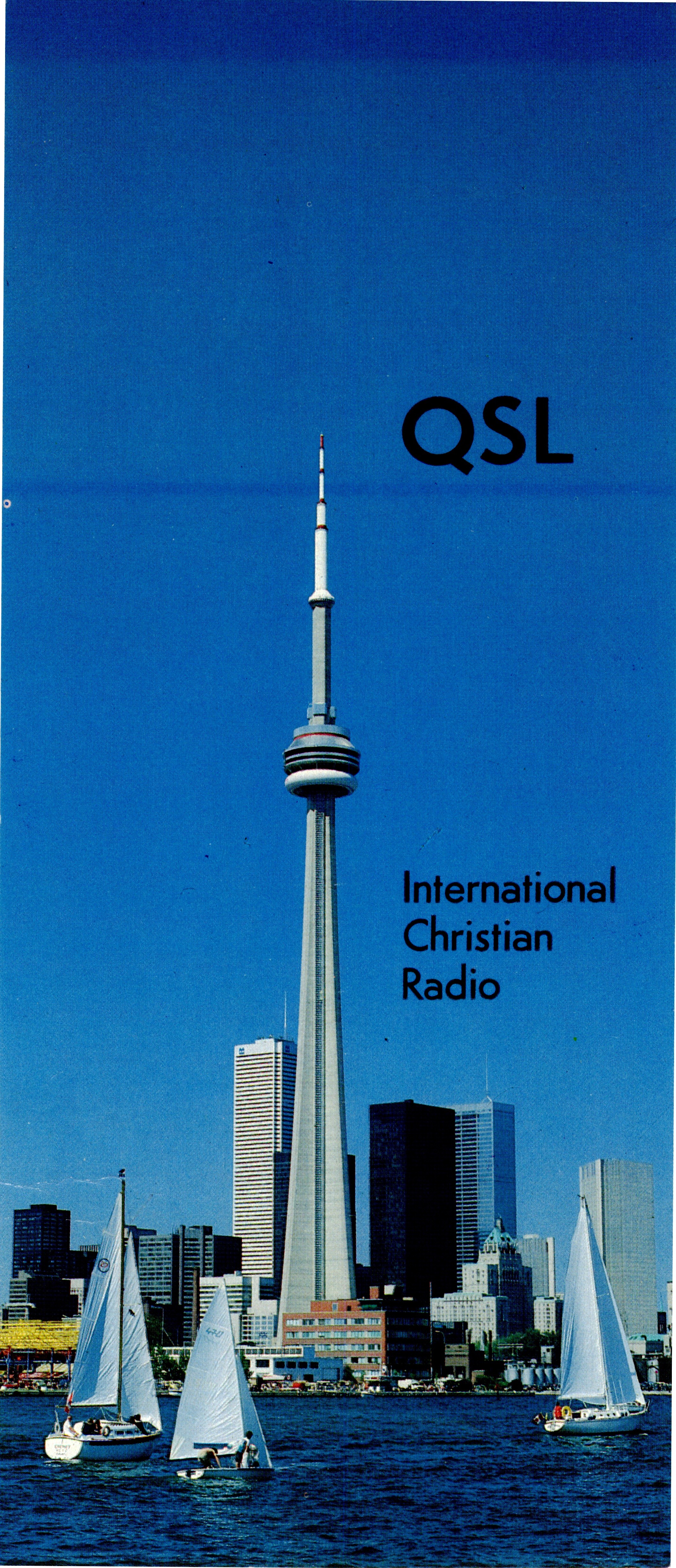The image is a tall, vertical advertisement showcasing a striking cityscape at the horizon line, with a rich dark blue body of water spanning the bottom section. Within the water, there are three sailboats: two on the left and one on the far right. The city is composed of various buildings; smaller brown and gray structures are situated in the foreground, while an array of tall, rectangular and square-shaped skyscrapers dominate the distant skyline. The centerpiece of the city is a towering spire that reaches almost to the top of the image. The spire features a wider middle section before tapering off to a pointed top. In bold black text at the top of the tower, it reads "QSL International Christian Radio," with "QSL" positioned slightly to the right. The sky in the background is a clear blue, hinting at a daytime setting. The image quality is slightly grainy, giving it an older, vintage feel.